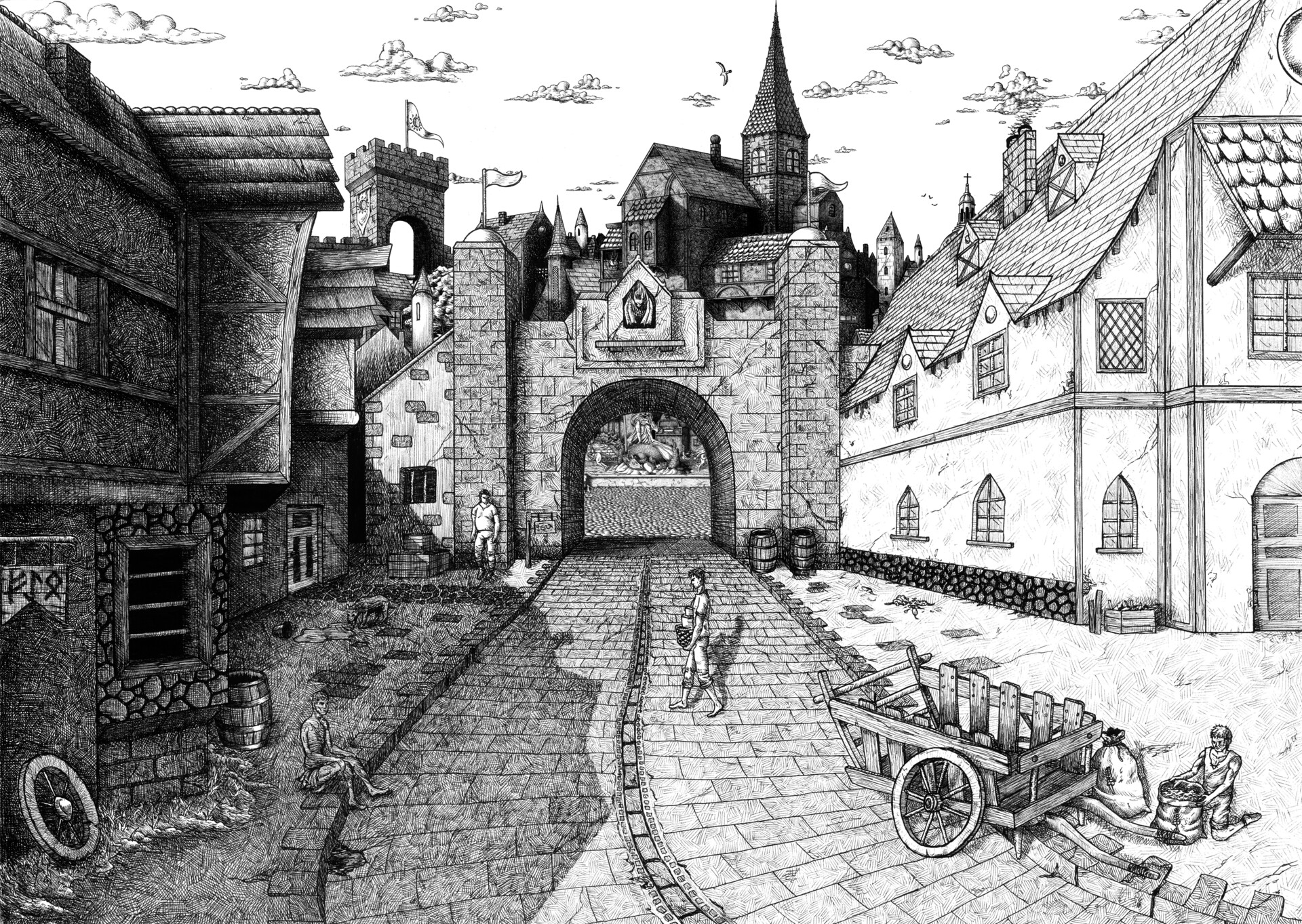This black and white drawing meticulously depicts a medieval scene, capturing a quiet moment in what appears to be a European village, possibly from Tudor-era England. Central to the image is a long stone-paved pathway leading through an arched brick gateway, which appears to serve as the entrance to a grand manor house or castle with a tall steeple. The sky above is bright white, adorned with puffy clouds and a solitary bird.

On the right side of the pathway, a prominent Tudor-style building with a white facade and dark wooden framing stands, its domed windows giving it a residential look. Closer to the viewer, in front of this building, is a crudely built wooden cart or wagon, where a man is kneeling, tending to a sack of goods, perhaps food or produce. To the left of the gateway, slightly shrouded in shadows, is a building that resembles a tavern, constructed primarily from stone, straw, and wood.

Scattered along the pathway, a few people engage in various activities. One person is standing while another, possibly carrying a basket, walks along the road. There is also a gentleman leaning against the entrance and another sitting by the roadside. Farther in the background, a small tower with a pointed roof and a visible flag adds to the castle-like ambiance of the scene.

The detailed line art showcases fine patterns and strokes, highlighting the textures of the brickwork, the wooden materials, and even the nuts and bolts on the wagon, enhancing the historical feel of this intricate and serene village illustration.